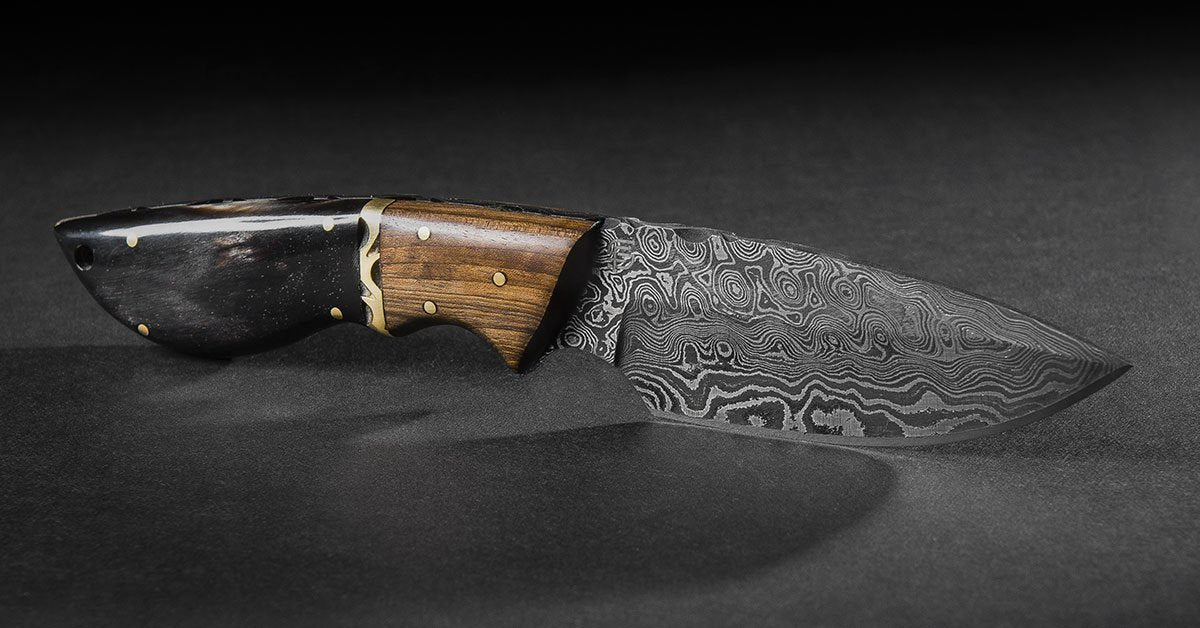The image depicts a knife positioned blade-down on a dark gray table, casting a shadow in front of itself, indicating the light source is from behind. The handle of the knife is intricate, featuring a multi-colored wood design: dark brown at the top transitioning to black at the bottom, adorned with what looks like small tan dots or rivets holding it together. The handle also includes decorative gold painting, adding to its ornate appearance.

The blade itself is a striking piece of craftsmanship, characterized by a series of swirling, whorled, and striated patterns in gray and white, giving it a water-like appearance. These patterns are not typical for most knives and suggest a hand-forged quality, adding to the blade's unique visual appeal. The composition highlights the detailed design and craftsmanship of both the handle and the blade, set against a simple dark background that emphasizes the knife's features.